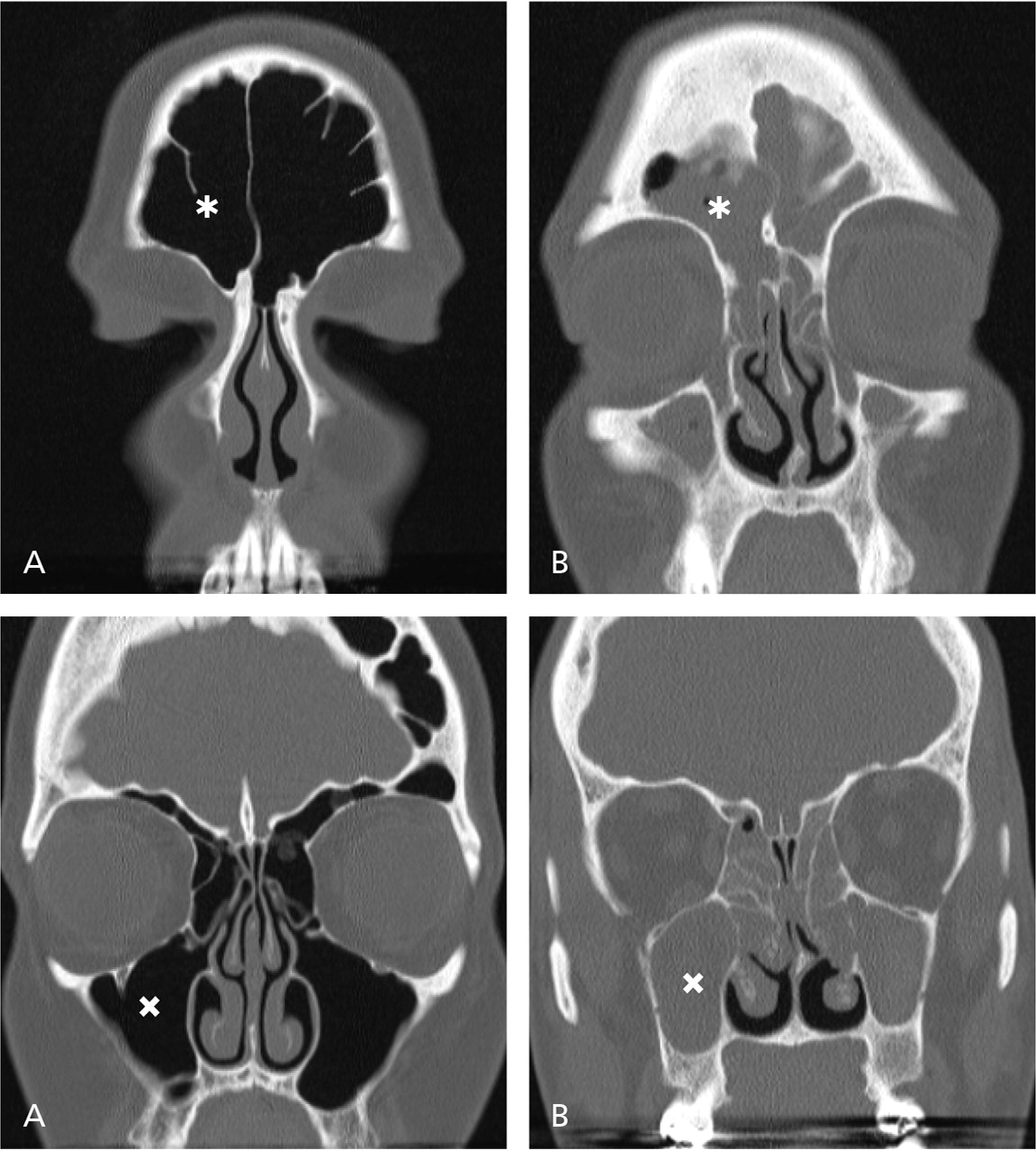This image displays a series of MRI scans, arranged in a grid of four sections, delineated by white intersecting lines forming a cross. Each section is labeled A or B and depicts different views and zoom levels of a human skull.

In the top-left quadrant (A), the grayscale scan provides an extensive view of the skull, showing a large black fan-shaped figure bordered by a white outline within a gray, blob-like structure. Adjacent to this, the top-right quadrant (B) offers a closer view, featuring detailed white highlights inside the gray structure and a smaller black area nearer the center. Both top images show an asterisk positioned on the left lobe, just above the eye socket.

The bottom row continues with further zoomed-in imagery. The bottom-left quadrant (A) reveals a larger, detailed white shape occupying the upper half of the skull and a prominent black shape in the lower half with gray detailing. Directly to its right in quadrant B, the image zooms in even closer, emphasizing the eye and nasal cavities, with only thin white shapes and minimal black areas visible. Both lower images include an X marking on the left side, beneath the left eye socket corresponding to the left maxillofacial sinus cavity.

Across all images, the scan evolves from an overall structure in quadrant A of the top row to highly concentrated anatomical details in quadrant B of the bottom row, elucidating various internal features of the skull.